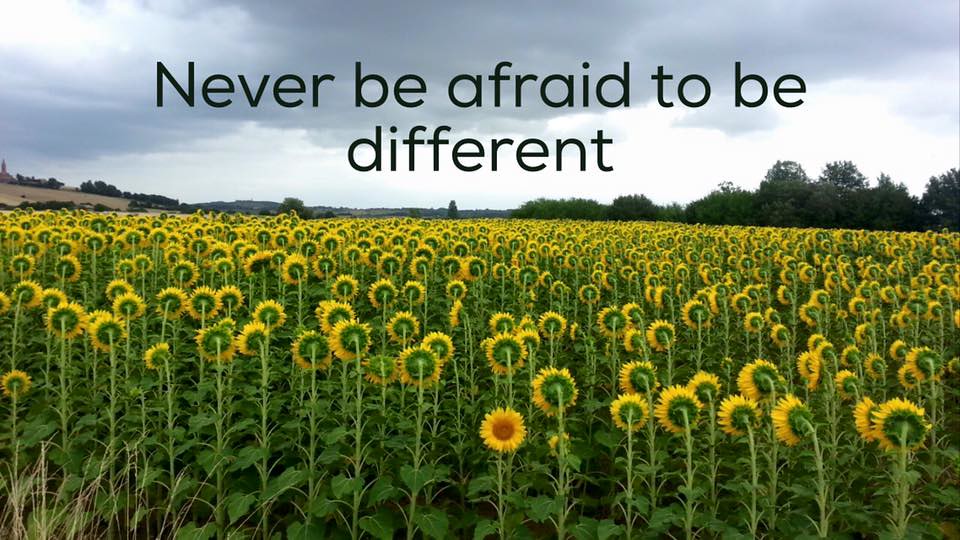The image is a picturesque, possibly CGI-generated, photograph of a vast field brimming with blooming sunflowers, which appear heavily altered. The field stretches to the horizon where stands of trees and a hill are visible. Under an overcast, gray sky filled with clouds, there is an inspirational quote in thin, bold black text reading, "Never be afraid to be different." The sea of sunflowers is uniformly facing away, except for one unique sunflower that directs its gaze toward the camera, embodying the quote's message. The scene's polished appearance and motivational caption suggest it is designed for social media, evoking a sense of encouragement and uniqueness amidst conformity.